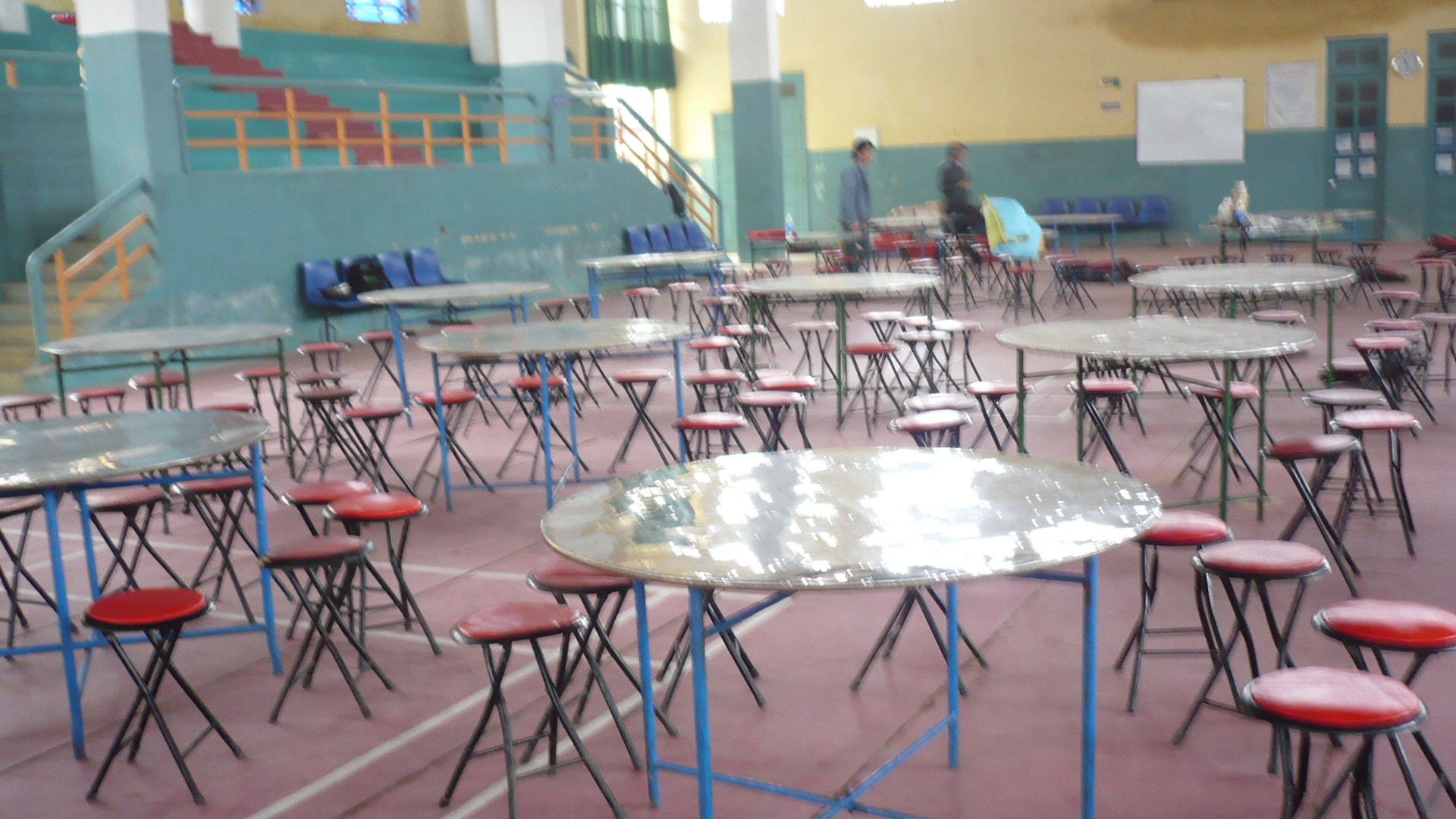The photograph depicts a large, somewhat blurry, indoor space, likely a school gymnasium or cafeteria, set up for an event. The image captures a spacious area with a red gym floor featuring various white sports markings. Scattered throughout the foreground are several rounded tables, each with shiny, reflective tops and blue metal legs, paired with stools that have black metal legs and red seats. There are approximately ten to eleven of these tables, each surrounded by multiple stools.

In the middle ground, there are visible stairs that are red in the center and turquoise on the sides ascending to a turquoise and white balcony supported by large pillars. The balcony is partially obscured but is accented with a yellow color towards the top. 

To the left, additional stairs also ascend from the floor. On the far right, a whiteboard hangs on the wall near two large turquoise doors with small square windows—one door more distinctly visible than the other. Near the balcony, two indistinct figures stand; one appears to be a male in a white jacket, while the other is a female dressed in black.

Overall, the image highlights an expansive, colorful, and multi-functional space with ample seating arrangements and vivid architectural features.